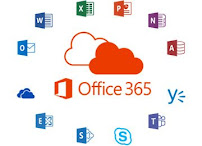A screenshot from Microsoft Office 365, displaying a collection of various application icons arranged in a circular layout on a white background. At the center, there is a prominent orange cloud overlapping a dashed outline of another cloud, also orange but not filled in. Accompanying the central graphic is an orange square next to the text "Office 365." Encircling this are multiple app icons: starting at the top and proceeding clockwise, there is an open folder with a "P" in a shade of orange-red, followed by a purple folder featuring an "N," a dark red folder with an "A," and a blue "Y" with three horizontal lines. Next is a blue folder marked with a "T," which also contains human figure icons, representing collaborative features. Continuing around, the icons include a Skype button, a blue folder with an "S," followed by a blue folder bearing an "E." Adjacent is a blue cloud icon and a blue folder showcasing an "O" with an envelope inside. The sequence finishes with a Microsoft Word icon represented by a blue folder with a "W," and a green folder labeled with an "X."